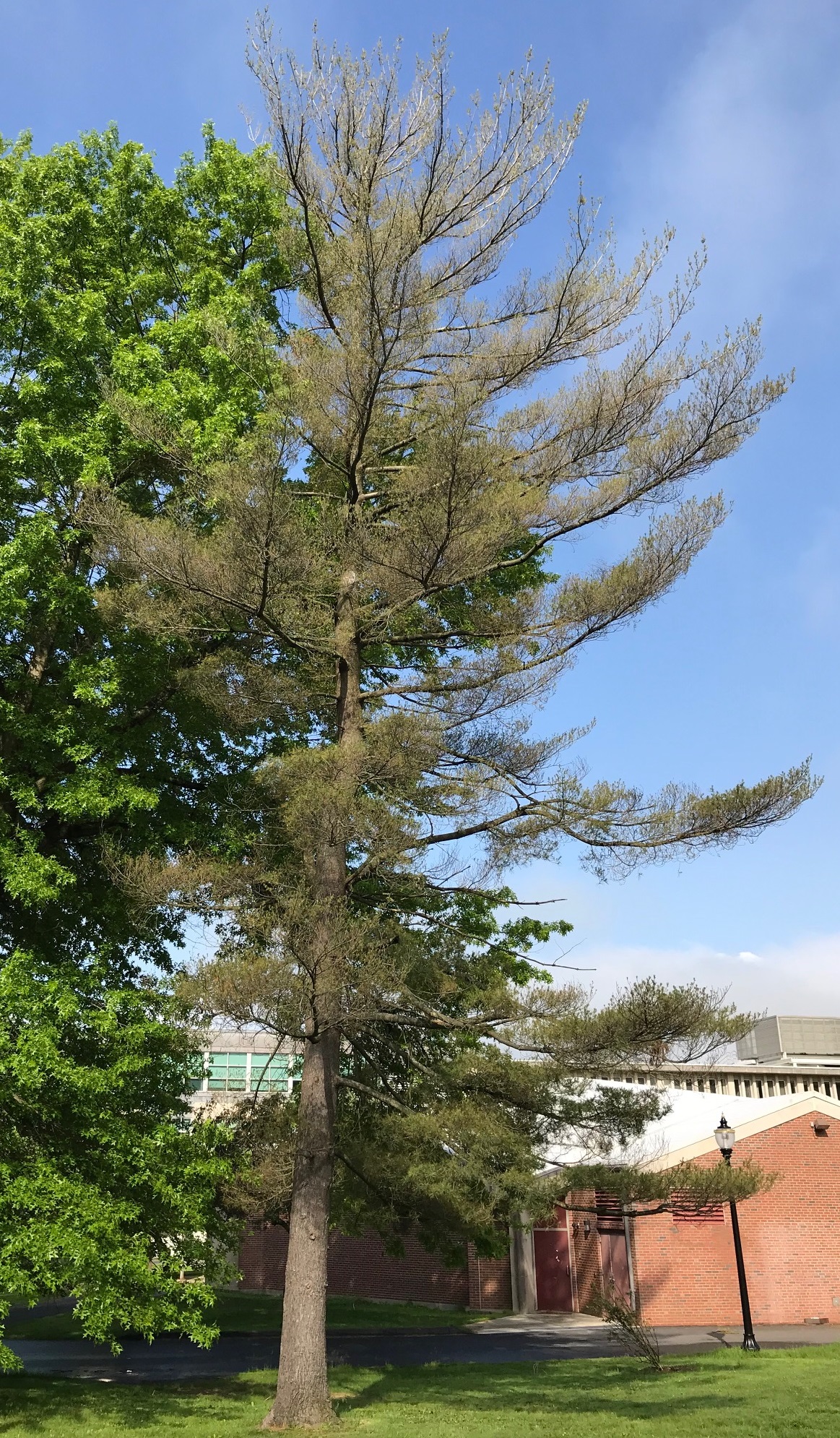The image is a tall outdoor scene centered around two trees on the left side. The tree on the far left edge of the image is lush and full of vibrant green leaves. Right next to it, slightly towards the center, stands a taller tree with a gray trunk, beginning to branch out about a quarter of the way up, adorned with sparse and dry, pale green leaves. In the background, towards the right, there is a one-story red brick building featuring a white roof and a red door, which evokes a school campus vibe. Adjacent to this building, there's an even taller structure with green windows. A distinct black lamppost with a cylindrical-shaped clear lens at the top is situated near the building. The foreground is composed of a green grassy area leading to a gray pathway, with wispy white clouds visible in the sky above.